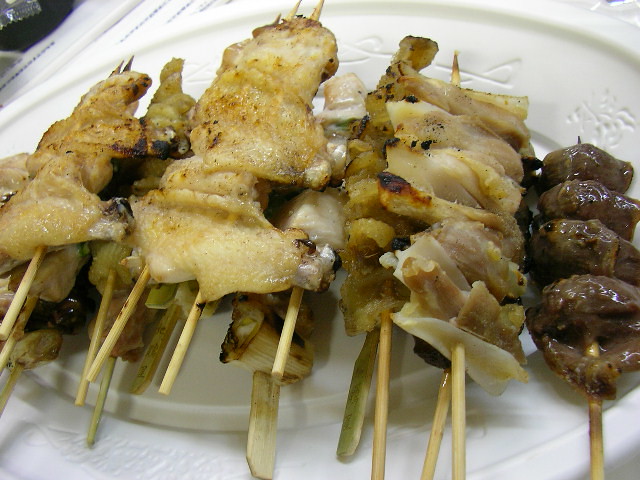The image features a variety of skewered foods, prominently displayed on what appears to be an oval white plate with some etching visible at the top. The skewers include an assortment of chicken and beef kebabs, totaling approximately 12 chicken skewers alongside 1 beef skewer. The chicken and beef pieces range in color from tan to dark brown, some slightly charred, providing a visually appealing contrast. A few of the skewers are garnished with melted cheese, adding a glossy sheen, likely from grease. Additional details, such as onions and potentially other vegetables like mushrooms or bacon, are interspersed among the meat skewers. The food occupies the majority of the frame, making it the main focal point of the image.